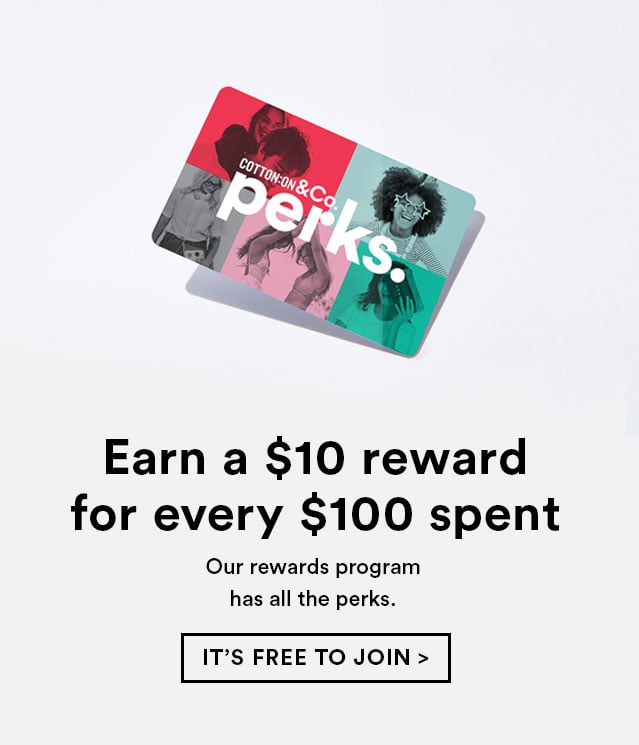The image is a screenshot of an advertisement set against a light gray background. At the top center, there is a picture of what appears to be a gift card or credit card. This card features white text that reads "Content on & Co Perks." Behind the card is a grid of five stylish, designer-like images, each overlaid with various colors to create a color-block effect. These images depict different people in dynamic poses, some featuring pairs and others individuals, possibly kids and young adults. The card is tilted upwards, casting a shadow to its left.

Below the card, centered text in large black font reads: "Earn a $10 reward for every $100 spent." This message spans two lines. Beneath this, another message reads: "Our rewards program has all the perks." also split into two lines and followed by a period.

Further down, there is a black rectangular outline containing capitalized black text that says, "IT'S FREE TO JOIN >", indicating a clickable button. This section contrasts with the smaller, sentence-case text above it.